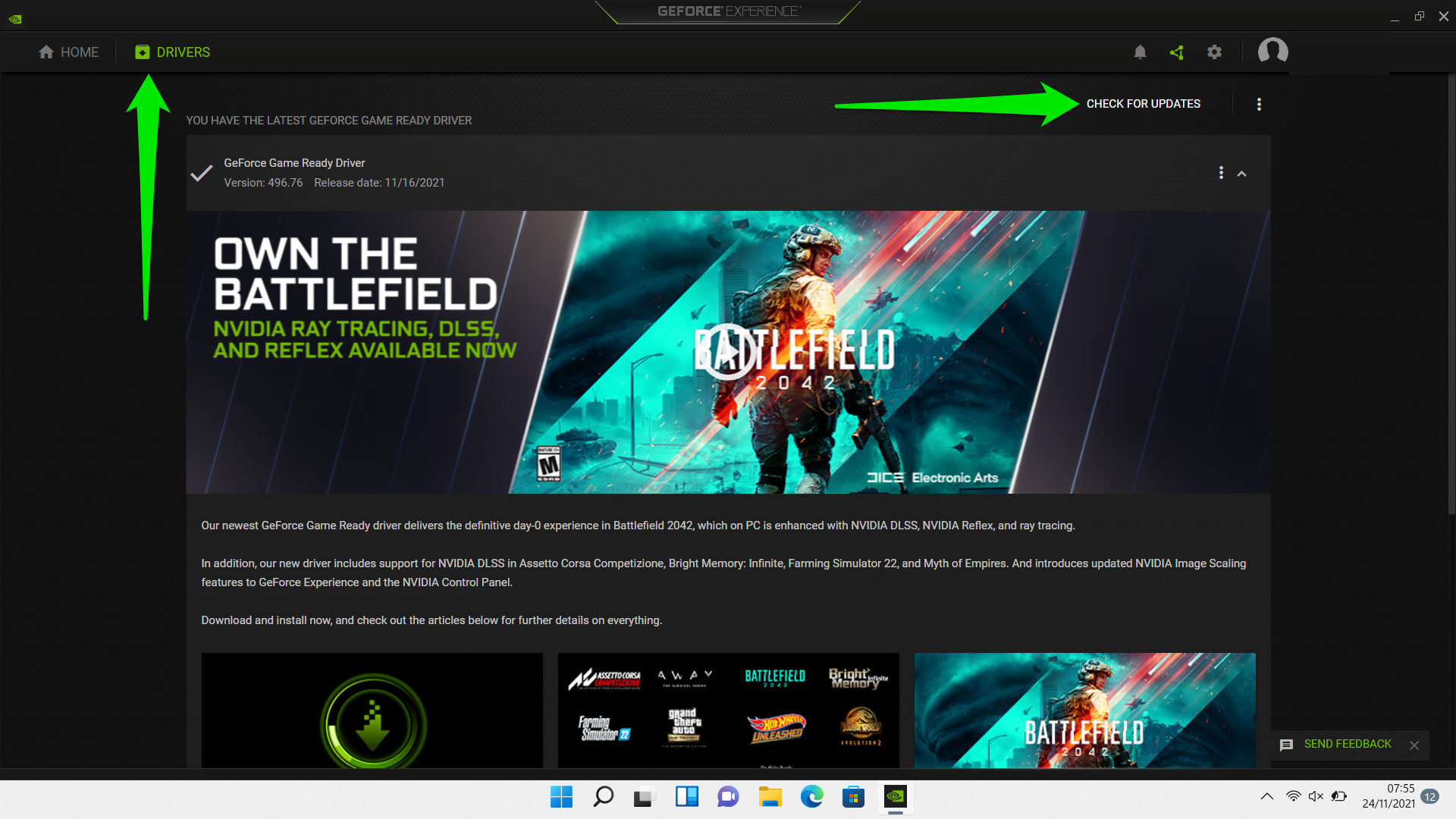This is a detailed screenshot of the GeForce Experience application, which manages the graphics card drivers for the computer. The app interface is predominantly black. In the top-left corner, it includes menu options labeled "Home" and "Drivers," with "Drivers" currently selected and highlighted in green. Directly beneath "Drivers," there is an edited green arrow pointing upward, emphasizing that this is the first option to click.

On the upper right side of the screen, there's a small white text that reads "Check for updates." Another green arrow, this one pointing rightward and situated to the left of the text, is edited onto the screenshot to direct attention to this button, indicating the second step after clicking "Drivers."

The main section of the screen features an advertisement for the game Battlefield 2042, which includes the text "Own the Battlefield, NVIDIA Ray Tracing, DLSS, and Reflex available now." Above this ad, there's a white check mark accompanied by the text "GeForce Game Ready Driver," along with the version number and release date of the driver. This screenshot serves as a guide, demonstrating how to check for updates in the GeForce Experience app step-by-step.